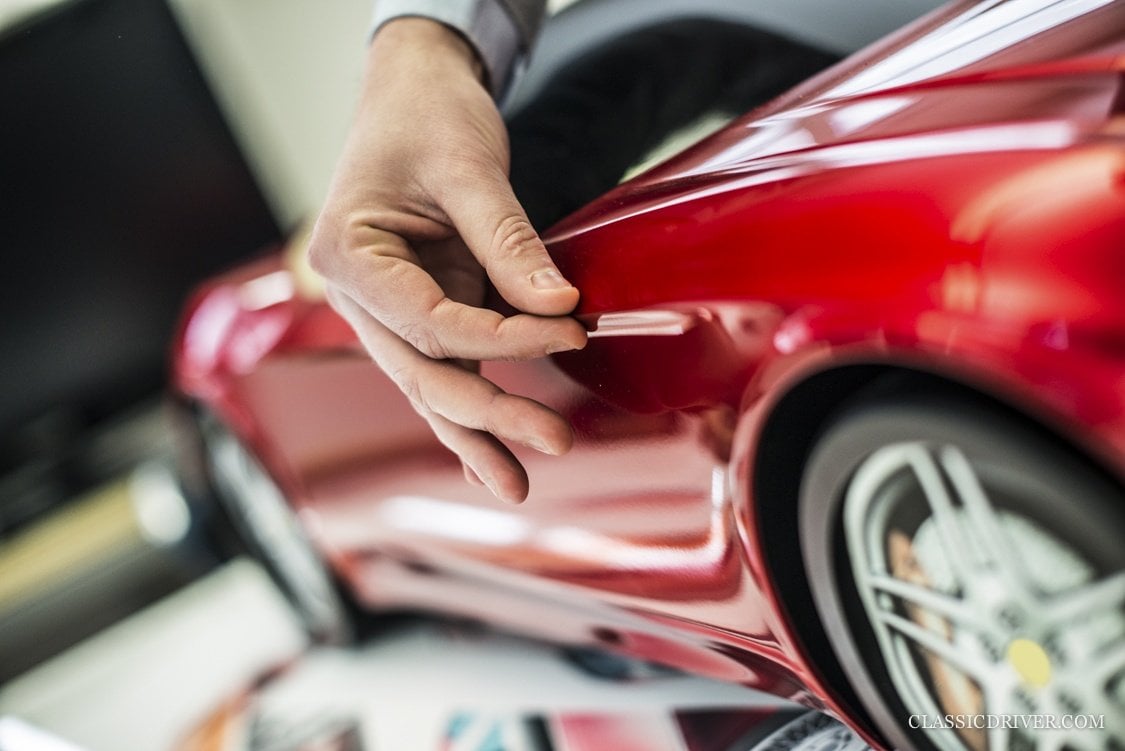In this detailed image, a Caucasian male's pale to light-toned hand descends from the top, with his thumb and forefinger pinched together, touching the side handle of a glossy red sports car, which might be a convertible. The angle of the shot makes the hand appear disproportionately large compared to the car, suggesting it could be a model rather than a full-sized vehicle. The background, along with the front and wheels of the car, is slightly blurred, focusing primarily on the hand, which is in sharp detail. The car rests on a white printed surface adorned with black, pink, blue, and orange designs. The male figure depicted in the image wears a long-sleeved gray printed shirt with a darker gray suit over it. Notably, the photograph features the website "ClassicDriver.com" written in bold white font in the bottom right corner.